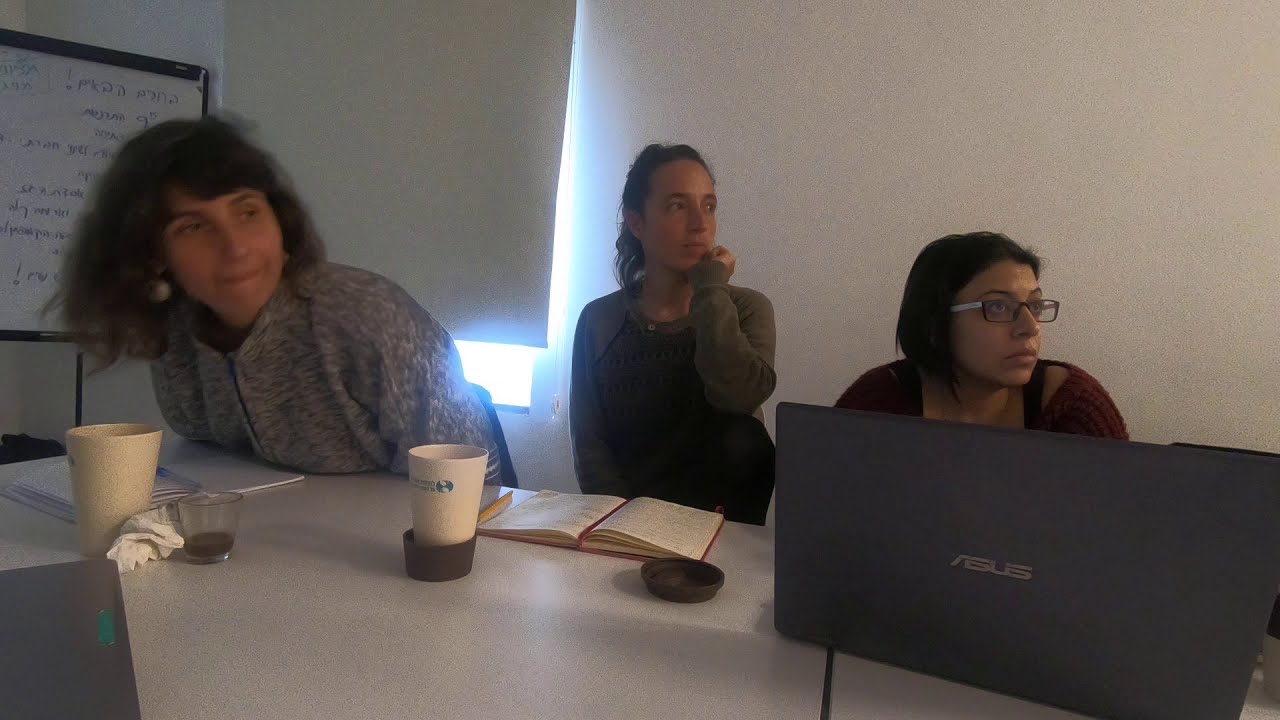In the photograph, a professional office setting is depicted, characterized by white walls and a conference table. Three women are seated at the table, unified in their attention to something off-camera on the right, suggesting a presentation or meeting. The woman on the far left has bushy brown hair and a cup of coffee beside her open paper notebook. In the center, the woman with tied-up dark hair also has a cup of coffee and an open notebook. On the right, a woman with glasses and black hair is positioned behind an Asus laptop. Behind them, a whiteboard with indiscernible, possibly foreign language words stands slightly obscured by the women. To the left of the whiteboard, a window with a partially lowered beige shade lets in blinding sunlight, contributing to the bright and open feel of the room. The ensemble of elements—the detailed focus of the participants, the informal office attire, and the array of utilitarian objects—paints a clear picture of a casual yet engaged work meeting.